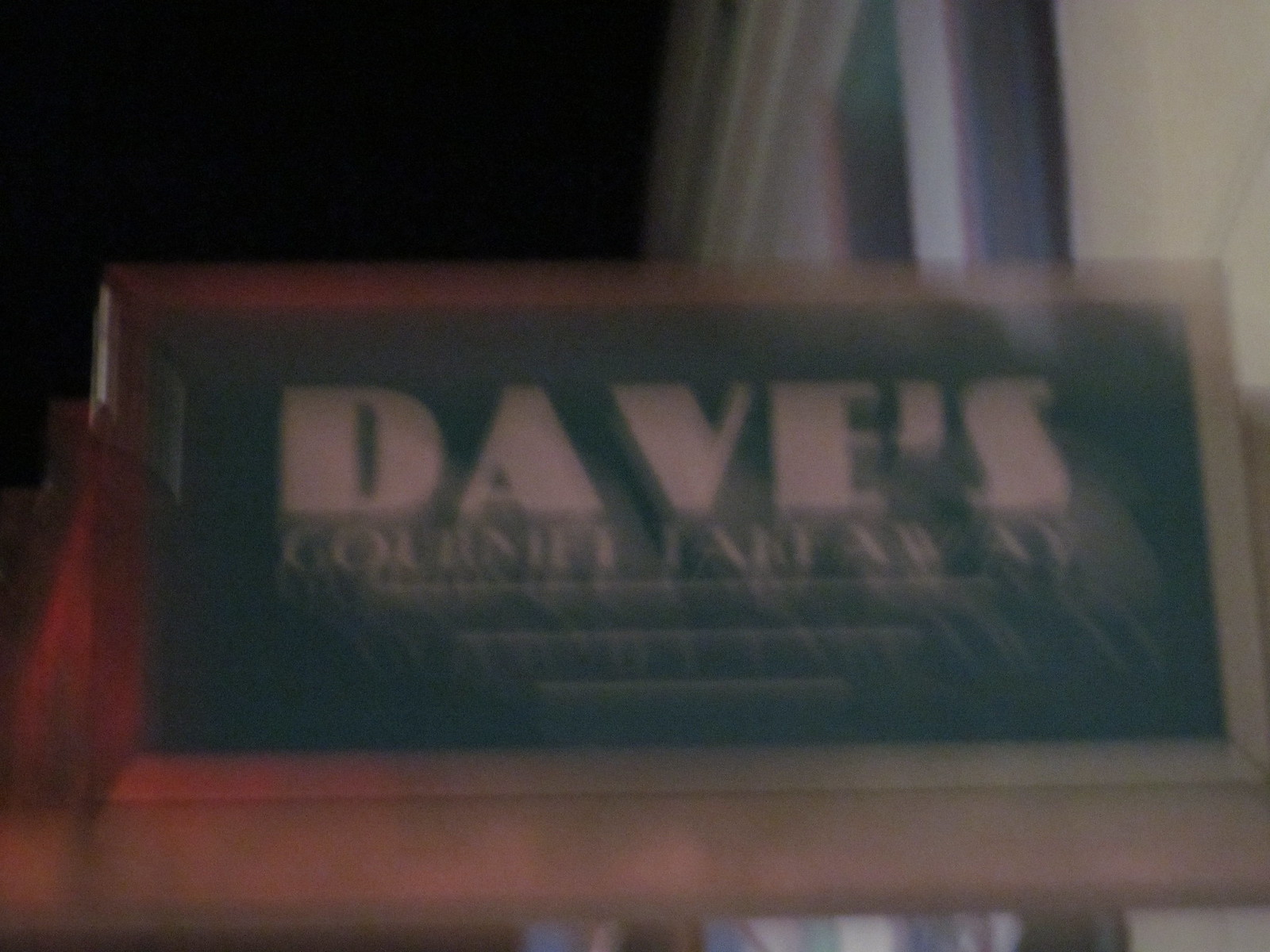A nighttime photograph capturing the exterior of a white building with multiple windows. The focal point of the image is a blurry sign, indicating that the photograph was taken while the camera was in motion. The sign, which is somewhat difficult to read due to the lack of focus, features a white border and a greenish-blue background. Prominently displayed are the words "Dave's Gourmet Takeaway," with "Dave's" written in bold, large white letters, and "Gourmet Takeaway" in smaller, thinner white text beneath it. The sign is affixed to the building, and the presence of a dark night sky in the top left corner accentuates the setting of the image.